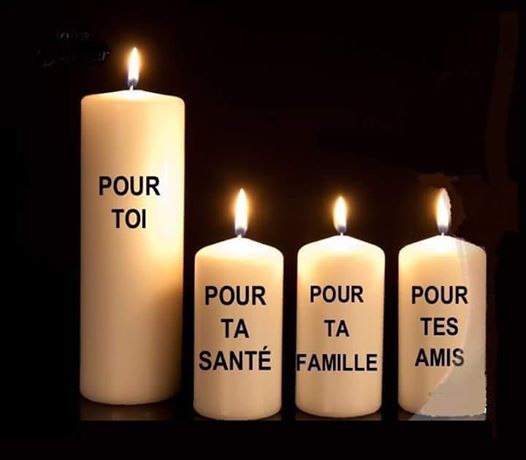This photograph captures a serene arrangement of four lit, off-white pillar candles set against an intensely black background. The tallest candle, situated on the left, is approximately twice the height of the remaining three. Each candle features blue French inscriptions in capital letters: the first reads "Pour Toi" (For You), the second "Pour Ta Santé" (For Your Health), the third "Pour Ta Famille" (For Your Family), and the fourth "Pour Tes Amis" (For Your Friends). The flames atop the candles glow with a warm yellowish-orange hue. The candles rest on what appears to be a brown table, though the darkness of the background makes it difficult to discern clearly. Furthermore, the candle on the left seems to be on a slightly raised platform, while the one on the right might be behind a glass enclosure, creating a frosted appearance near its base.